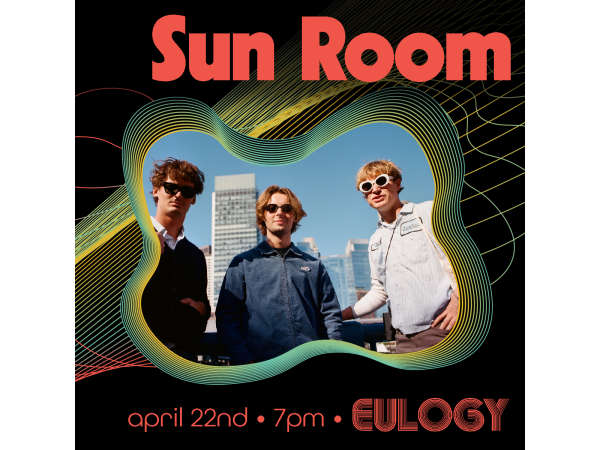This illustration serves as an advertisement for an event, prominently featuring a central photograph of three men with a cityscape background of tall buildings and a blue sky. All three men are wearing sunglasses, with the man on the left in a buttoned white shirt and sweater, the man in the middle clad in a denim jacket, and the man on the right donning a white shirt with a label on the chest. The graphics surrounding the photo are vibrant and psychedelic, dominated by black, yellow, red, and green stripes and curved lines, evoking a retro, old-school vibe. The text on the advertisement indicates several key details: the words "Sun Room," likely the event location or the name of the band, appear at the top in bold red. Additionally, the name "Oology" or "Eulogy" is prominently displayed, possibly referring to a band or DJ performing at the event. The date, April 22nd, and the time, 7 pm, are also clearly indicated within the colorful and dynamic design.